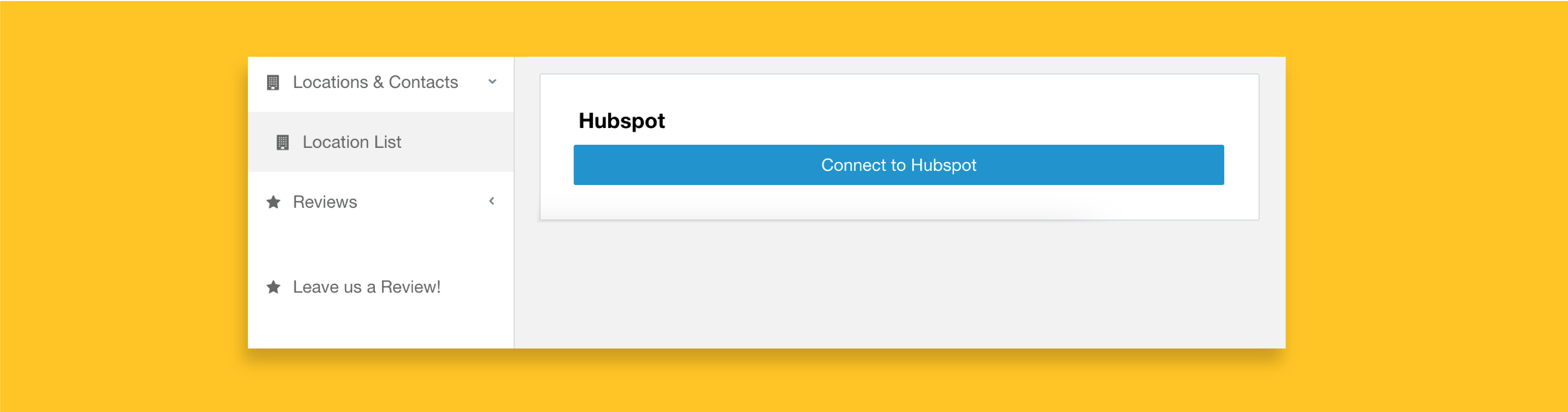This image is a cropped screenshot featuring a user interface overlaid on a yellow background with a subtle shadow effect. On the left side of the interface, there is a column with various dropdown options including "Locations and Contacts" and "Reviews." The "Locations and Contacts" dropdown is expanded, showing a selected "Location List" option highlighted in light gray. 

On the right side, the interface prominently displays "HubSpot" as the title, accompanied by a blue "Connect to HubSpot" button. The background of the HubSpot window is light gray, with the title and button encased in a clean, white rectangle. The overall design of the interface is simple and not in dark mode, characterized by muted colors and a straightforward layout. The screenshot is wide and thin, suggesting a minimalistic design approach. The operating system used is not identifiable from the image.